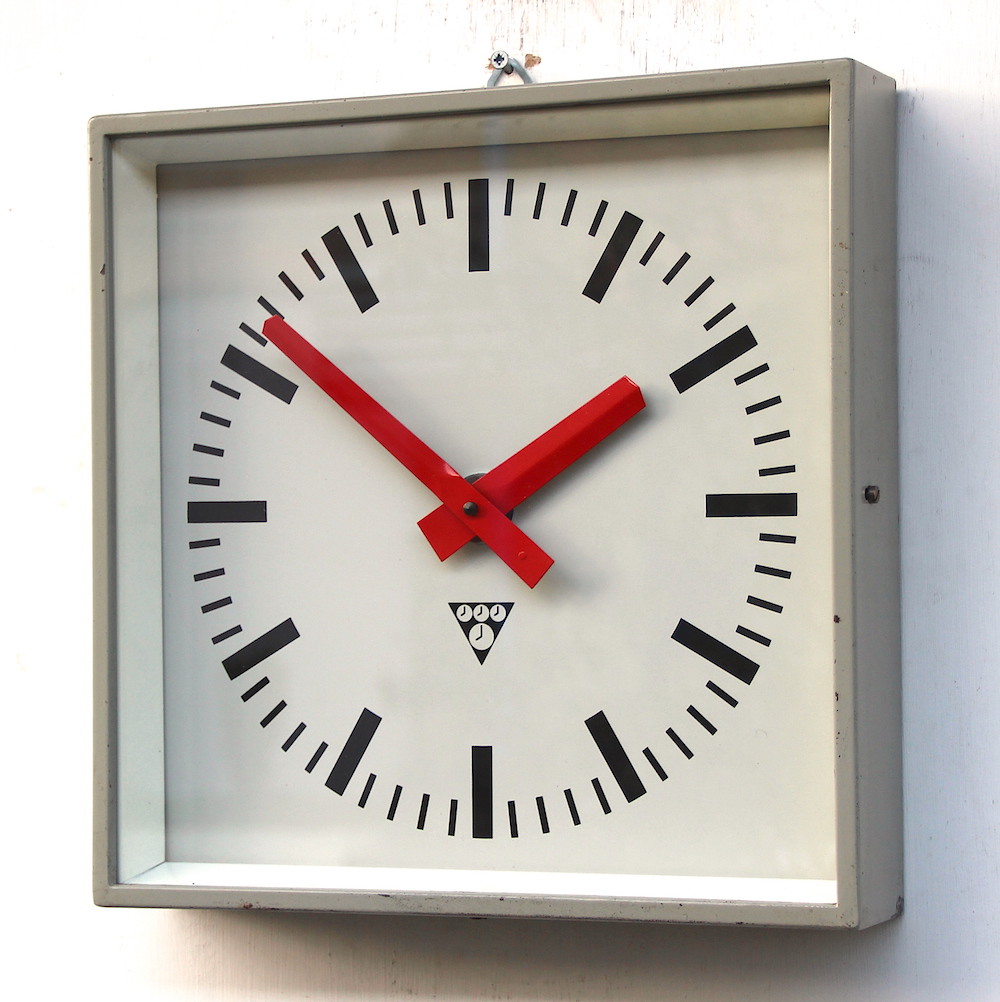This photograph captures a square analog wall clock mounted on a plain white wall. The clock, made of brushed stainless steel, gives off a modern and sleek aesthetic. It is suspended from a single exposed screw, showcasing its minimalistic design. The clock face is stark white, adorned with black rectangular dashes that denote the hours and minutes, lending to its contemporary style. The hour and minute hands are also crafted from metal and are painted a vibrant red, providing a striking contrast against the monochromatic face. Notably, a triangular clock symbol is positioned at the bottom of the clock face. The time displayed is 1:52.